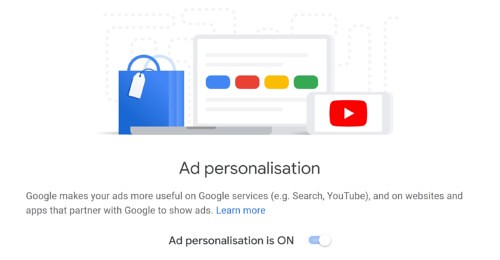A detailed description of the screenshot of the Google-related image could be:

---
The screenshot features a visually appealing design representative of Google services. Central to the image is an illustration, either drawn or rendered as vector graphics, of a blue shopping bag resembling a paper bag. Adjacent to this, there's a stylized laptop displaying four consecutive ovals in Google's signature colors: blue, red, yellow, and green. Additionally, the familiar YouTube logo is present, characterized by a red rounded square or rectangle with a white play button triangle in the center.

Beneath these visuals, the heading reads "Ad Personalisation," with the spelling indicating either Canadian or UK English usage (P-E-R-S-O-N-A-L-I-S-A-T-I-O-N) in a bold black font. Following this, there's an explanatory text in black stating, "Google makes your ads more useful on Google services, e.g. Search and YouTube, and on websites and apps that partner with Google to show ads."

Towards the end of the description, there's a blue hyperlink labeled "Learn more." Finally, it confirms the status of the feature with the phrase "Ad personalisation is on," marked by a check symbol.